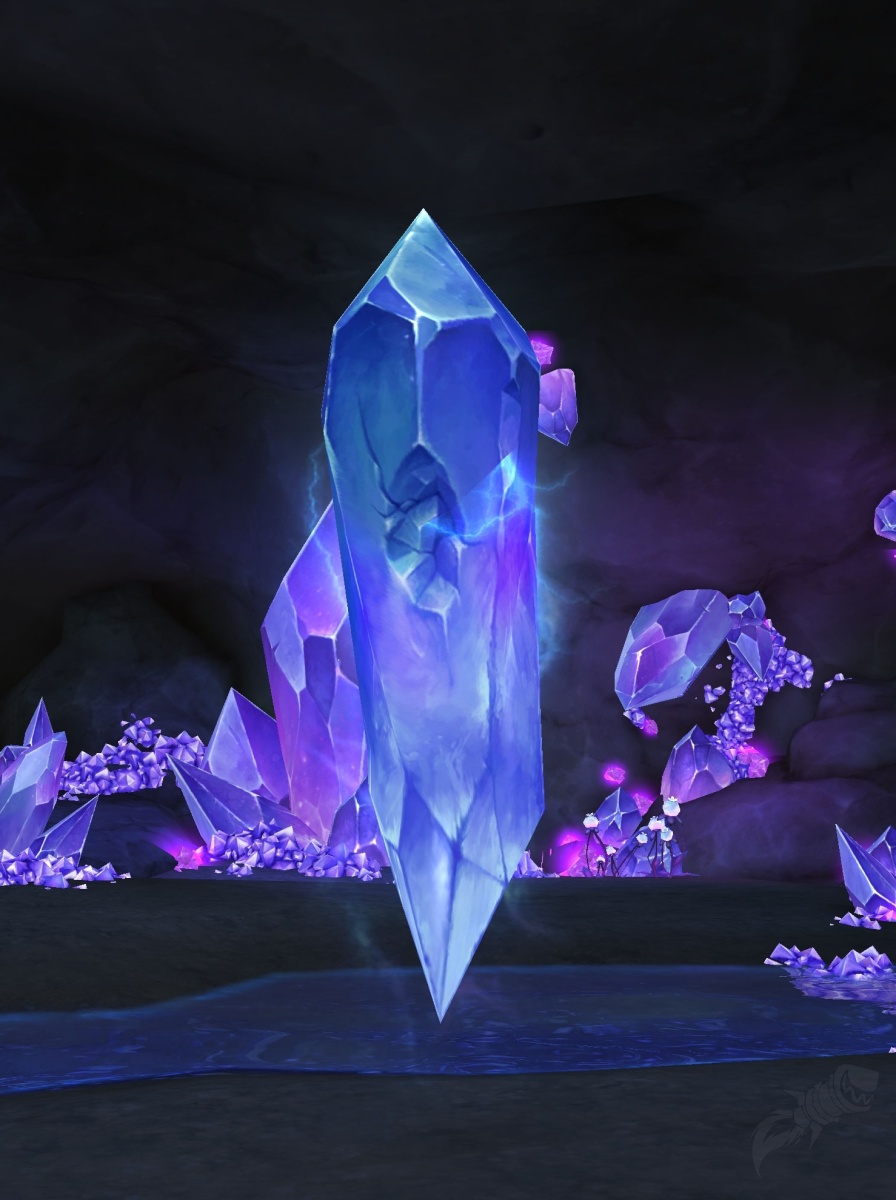This image depicts a surreal, artistically rendered crystal cave. The backdrop is composed of dark black and gray rock, extending vertically and creating a cavernous atmosphere. Dominating the center of the picture is a large blue crystal shard, standing vertically on one of its sharp points. This central crystal features a distinctive crack or chip on its front, adding texture and intrigue. Surrounding the main crystal are numerous smaller clusters of crystals, primarily in shades of purple and blue, varying greatly in size, from tiny fragments to larger, more defined forms. These crystals are scattered across the ground, enhancing the ethereal ambiance of the cave.

Beneath the central crystal and traversing the bottom of the image is a dark blue strip, resembling a small creek or stream, though it maintains an abstract quality making it possibly another geode or a reflective surface. This bluish element adds a contrasting splash of color against the otherwise dark and mysterious cave floor. The smaller crystals alongside create a dynamic visual with their translucent bodies catching and reflecting light, suggesting that they might be the only source of illumination within this mystical underground setting. The overall composition creates a fantastical, almost otherworldly scene that blurs the line between reality and imagination.